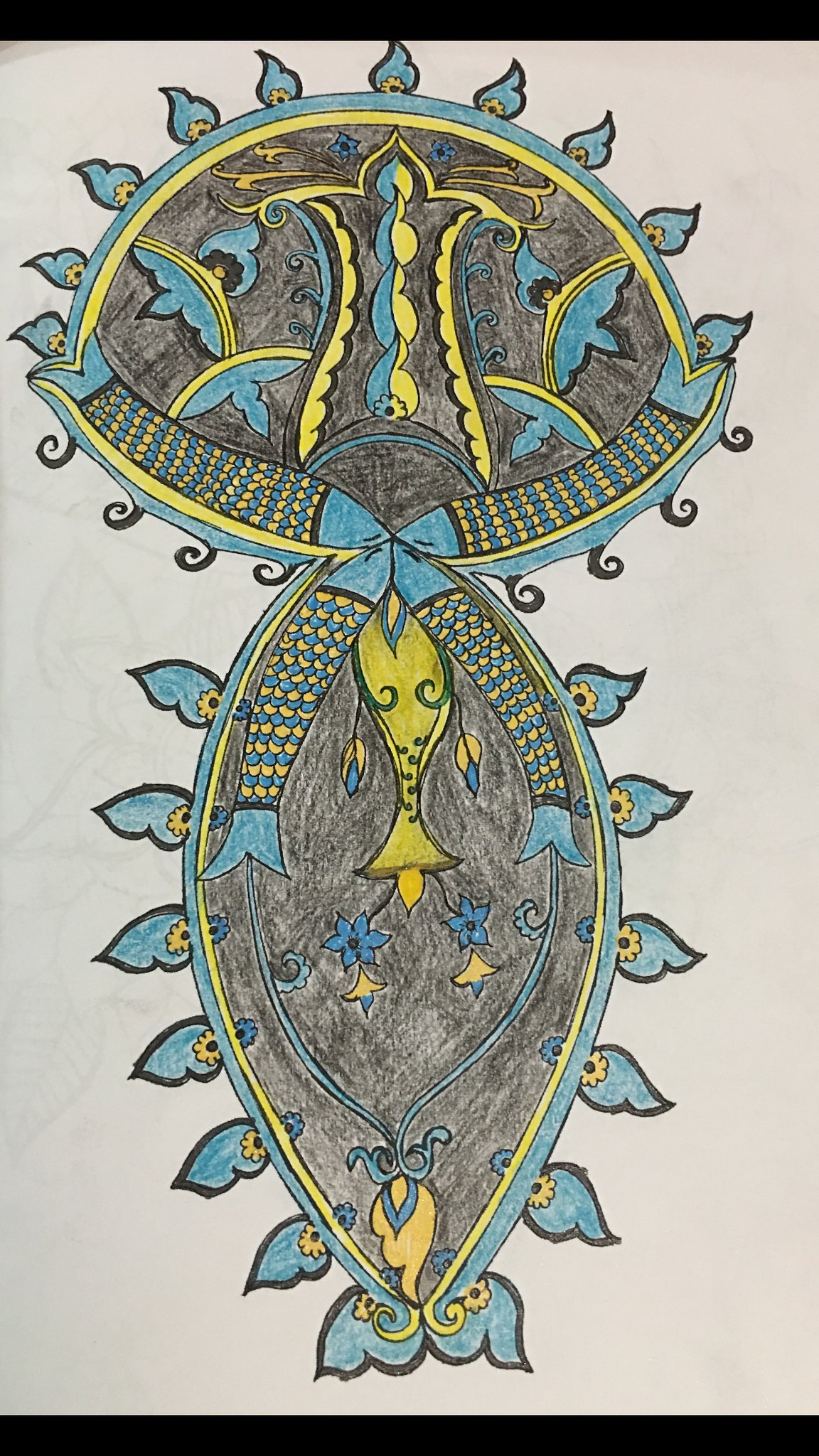The image is a detailed drawing on a white piece of paper, resembling a mandala but centered around a character-like figure. The top portion of the drawing features a horizontally-oriented oval, outlined in light blue with a strip of yellow inside, filled with a brown-gray center. This oval represents a head with two intricate eyes and intricate patterns. The head has curly black lines at the bottom and blue flame-like designs emerging from the top.

Connected vertically below is another oval symbolizing the body, colored similarly with a vertical axis. The lower segment of this oval features two fish connected by their mouths. These fish are rendered in blue, yellow, and black, maintaining the drawing’s intricate and layered design motifs. Flower designs and additional flower motifs are scattered throughout the pattern, adding to the complexity. The overall color scheme includes black, blue, yellow, and occasional green highlights around squiggly lines. The photograph is framed by a black rectangular band at the bottom, suggesting the drawing is placed on a black surface, possibly within a coloring book as hinted by other floral motifs peeking from the side.